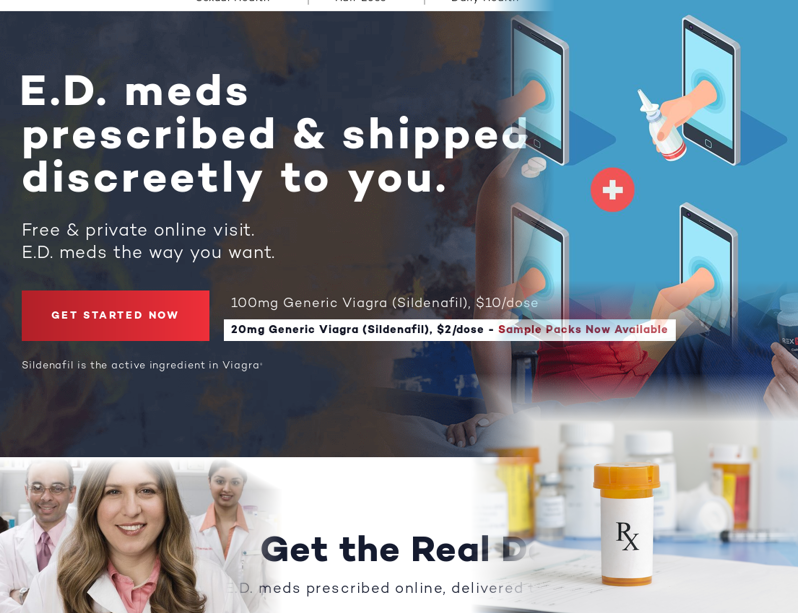This is a detailed caption for an advertisement image on a website for erectile dysfunction (ED) medicines. 

---

The advertisement prominently features information on ED medication available through the website. At the top, in bold white text, the website reads "ED meds prescribed and shipped discreetly to you." Beneath this, it offers a "Free and private online visit" with the tagline "ED meds the way you want." A call-to-action is evident with the phrase "Get started now" displayed in smaller white letters against a red background.

The image provides pricing information, noting that 10 or 100 milligrams of generic Viagra costs $10 per dose, while 20 milligrams of generic Viagra is priced at $2 per dose. Sample packs are also advertised. 

The background features a creative design, showing four images of a phone. It illustrates a user ordering the medication, with a hand physically reaching out of the phone, signifying the process of receiving the medicine. 

A highlighted statement at the bottom reads, "Get the real ED meds prescribed online delivered to you." This section also displays pictures of three pharmacists, alongside images of prescription medicine bottles and a syringe, symbolizing professional pharmaceutical services. The entire advertisement occupies the full screen, except for the segment showcasing the pharmacists and medicines at the bottom.